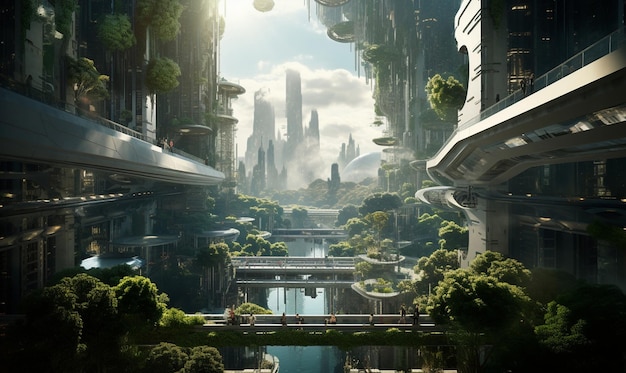The image depicts a futuristic, sci-fi cityscape designed with advanced conceptual architecture, seemingly crafted with digital tools like Photoshop. Two towering, silver-colored buildings stand prominently on the right and left sides, dimly lit, casting shadows towards the periphery. They are adorned with lush hanging gardens on various balconies and interconnected by multiple walkways and bridges, crossing over a pristine blue waterway. In the lower frame of the image, these bridges, shaded in parts, support walkways where people stroll, possibly heading towards pavilion-like areas below that may house restaurants surrounded by greenery. In the distance, the scene expands into a sprawling cityscape with tiers of skyscrapers that ascend from smaller to gigantic structures that pierce the bright blue sky, adorned with white clouds. A giant dome is visible to the right in the background, and rays of sunlight illuminate part of the cityscape, creating a play of light and shadow. Additionally, a fountain spraying water can be seen in the middle distance, further adding to the city's vibrant and thriving ecosystem.